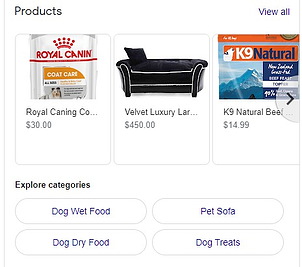This image is a cropped screenshot from a product section on a website, likely Amazon, displayed against a white background. The cropped area appears as a small square. In the upper left corner of the box, "Products" is written in small black letters, while towards the upper right side, there is an option labeled "View All" in tiny blue letters. Below these headings, the top section of the box showcases three thumbnail images of various products. Under each thumbnail, there is a partial text representing the product name, with the corresponding price listed directly below on the left side.

To the right of the thumbnails, a transparent semicircle contains a right-pointing arrow, indicating the option to scroll through additional product images. 

At the bottom of the cropped section, "Explore Categories" is written in small black letters near the left side. Below this text, there are four circular buttons (bubbles). The two bubbles on the bottom left are labeled "Dog Wet Food" and "Dog Dry Food," while the bubbles on the right are labeled "Pet Sofa" and "Dog Treats."

On the extreme left and right edges of the screenshot, faint gray lines are visible, marking the boundaries where the image was cropped.